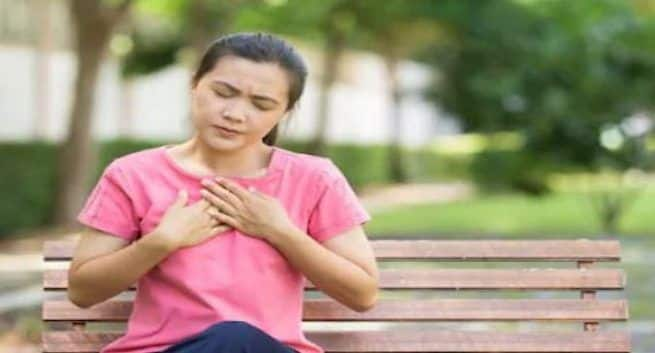The image depicts a woman sitting alone on a wooden park bench, gripping her chest with both hands and tilting her head to the right, suggesting discomfort or chest pain. She has brown hair tied back in a ponytail and is wearing a short-sleeved pink shirt along with blue pants that are partially obscured. Her eyes are closed, and her expression indicates suffering. The background showcases a natural park setting with green, healthy grass and trees, a dirt walking path, and bushes lining the left side of the path. Additionally, a blurry white wall can be seen behind the bushes. The image quality appears compressed with noticeable JPEG artifacting around the woman and the bench.